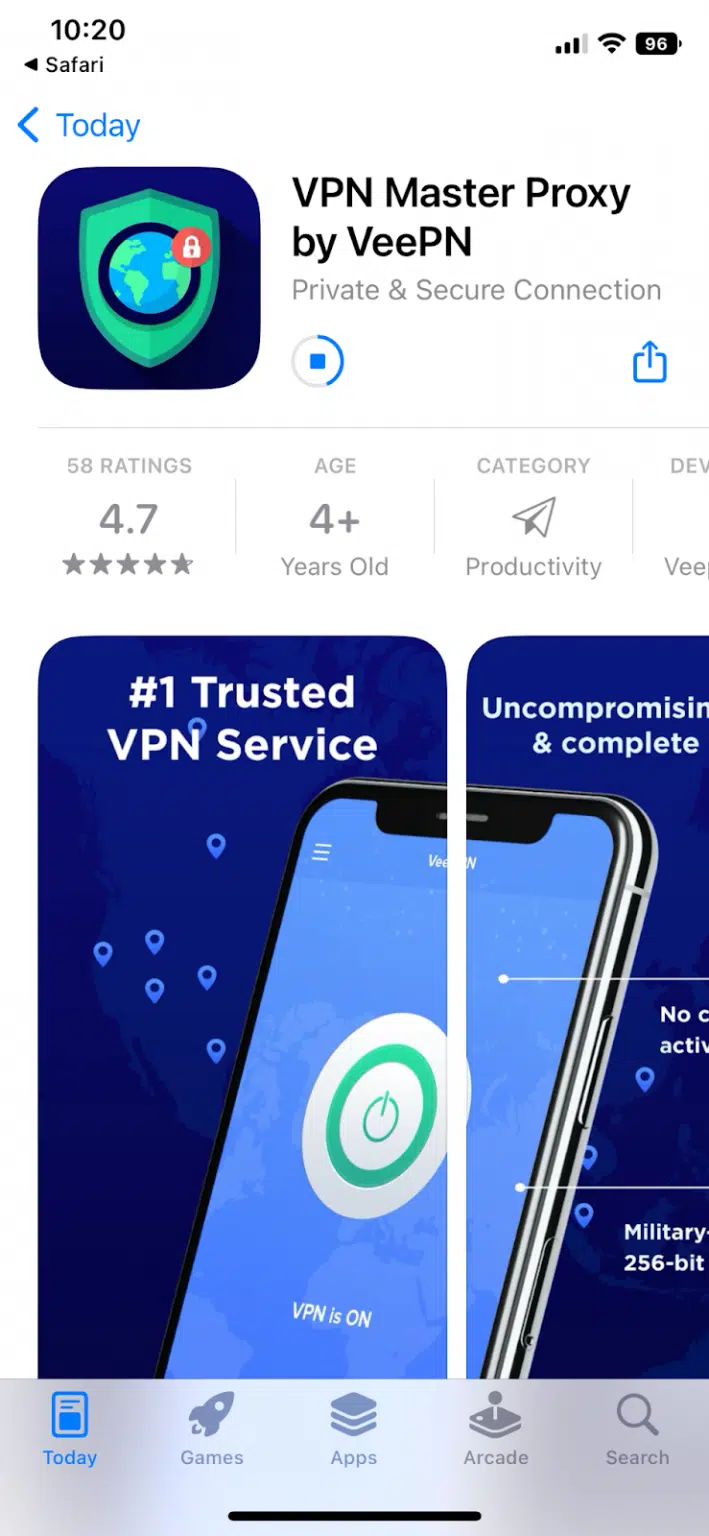Screenshot of the Apple App Store page for downloading "VPN Master Proxy" by VEE Group. The app is in the downloading phase, indicated by a blue progress ring that is approximately halfway full. To the right of the progress ring, a forward symbol is outlined in blue. The app's icon is displayed to the left, featuring a green shield with a black-outlined globe, a small red circle in the upper right corner, and a white lock on a deep purplish-blue background. Beneath the app's title, "VPN Master Proxy by VEE Group - Private and Secure Connection," the app boasts 58 ratings with an impressive average of 4.7 stars. It is rated suitable for users aged 4 and older and categorized under Productivity. Additionally, the screenshot includes segmented advertisements for the app, one of which proclaims it as the "Number One Trusted VPN Service."